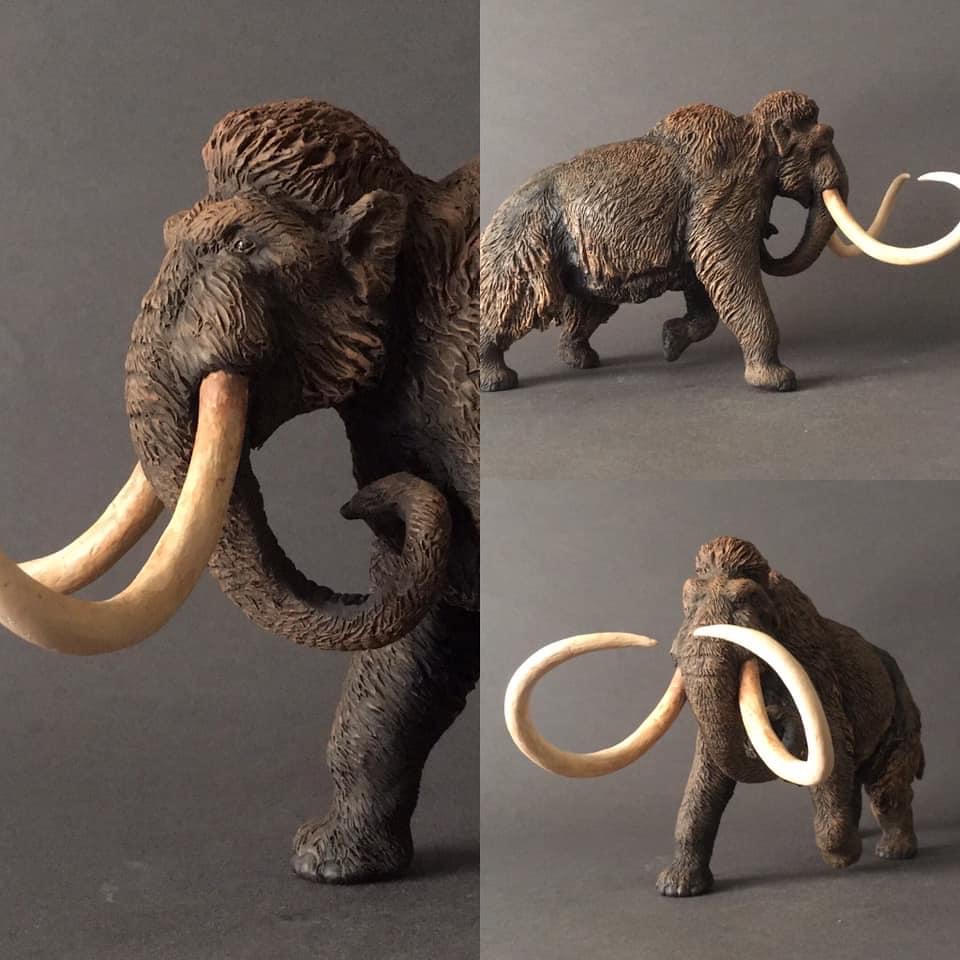The image showcases a detailed and expressive statue of a woolly mammoth, presented through three distinct photos merged into a single composite. The background is a plain brown, giving emphasis to the mammoth without distractions. The left image is a close-up of the mammoth's face and chest, highlighting its expressive features and one of its large, curved tusks. The top right photo provides a profile view, showing the mammoth with its left front leg extended forward, creating an impression of motion, as if it’s walking or charging. The bottom image presents a frontal perspective, capturing the mammoth advancing towards the camera with its right leg in the air. All images emphasize the mammoth’s long, curved tusks that nearly touch at their points, its thick fur, and a distinctive tuft of hair on its head. The statue’s fur and physical details suggest a lifelike representation, though the actual size remains uncertain without context. This could be a museum diorama or a model, but the impressive detailing captures the essence of the ancient creature vividly.